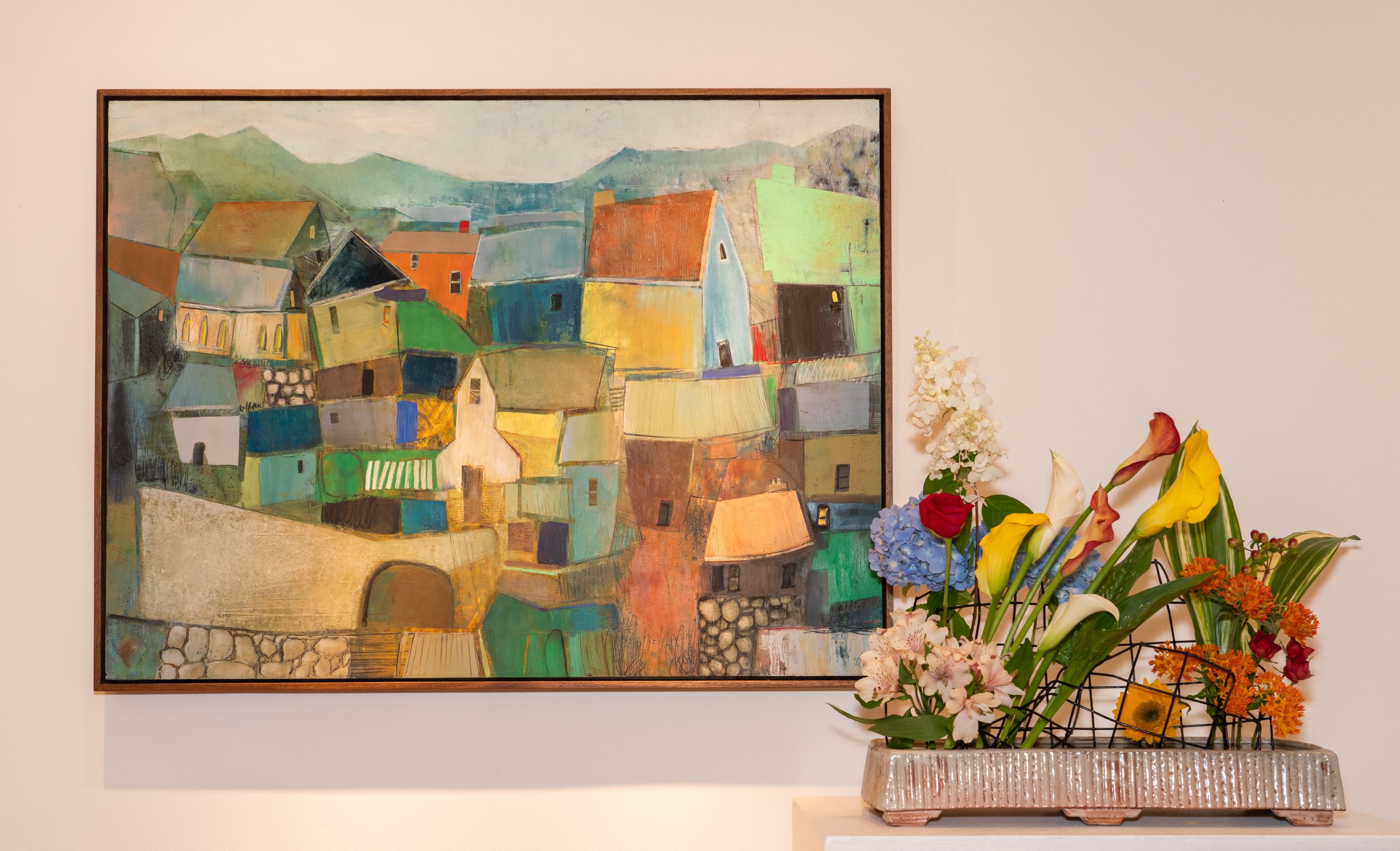The photograph features a distinct and vibrant scene dominated by a pink wall. Mounted on the left side of the wall is a striking painting enclosed in a thin brown wooden frame. The painting, suggestive of an abstract or impressionist style, depicts a colorful village with variously shaped homes – trapezoidal, square, and other forms – in a spectrum of hues including orange, blue, and green. The village is set against a backdrop of rolling hills or mountaintops, with some cobblestone walls incorporated into the scenery.

On the right side of the image, partially visible, is a light pink table. Atop this table rests a large tray of matching light pink color, holding a diverse array of flowers and foliage. The flowers are assorted in colors, showcasing shades of light pink, light orange, yellow, red, and blue, alongside green leaves. Identifiable among the floral assortment are a rose and a sunflower, with other species such as tulips and orchids suggested. The flowers appear to be supported by wires, adding structure to the arrangement. The setting is bathed in an overhead amber-colored light, highlighting the intricate details of both the painting and the floral display.